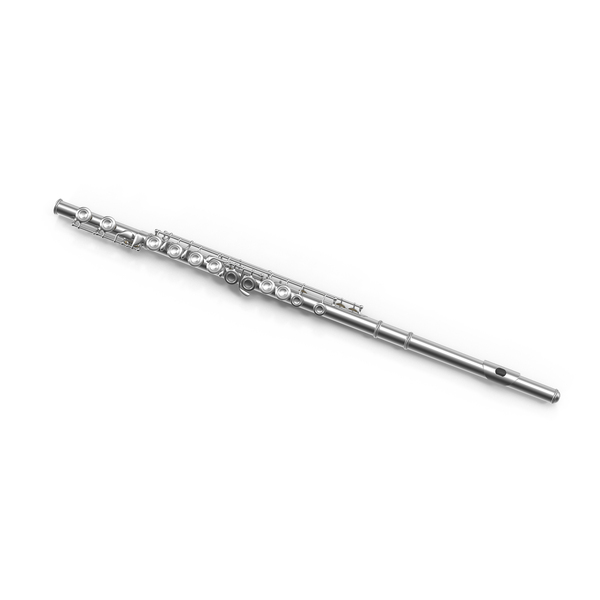This is a detailed product image of a standard metal flute, displayed against a white background. The flute, polished silver in appearance, extends diagonally from the higher top left corner to the lower bottom right corner of the image. The instrument resembles those commonly used in marching bands, with its long, thin, cylindrical shape akin to the diameter of a pencil. At the top left, the mouthpiece is visible, leading to a series of circular keys designed for finger placement. These keys, some facing upwards and others towards the side, run along the length of the flute. At the bottom right end, there is an open hole, presumably for sound projection. This detailed presentation highlights the intricate design and polished finish, typical of product images found on storefronts like Amazon.